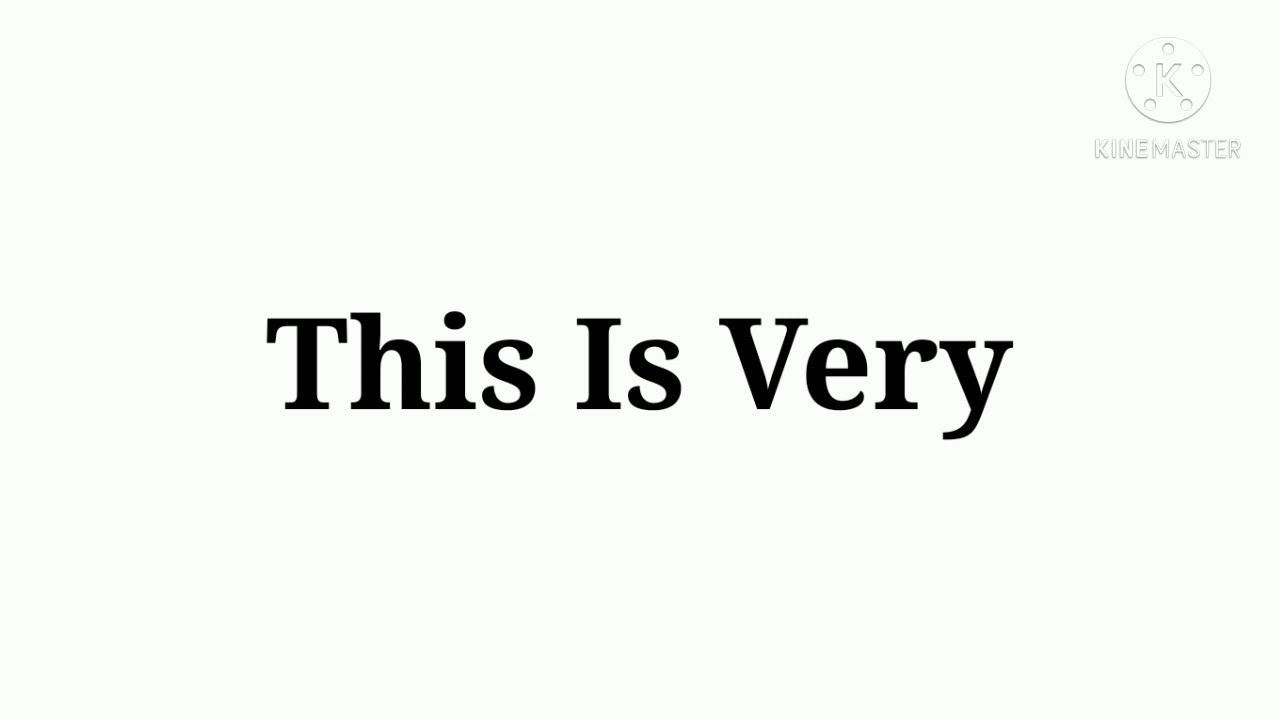The image features a slightly off-white background with the phrase "This Is Very" prominently displayed in black text at the center. The words are styled with capitalized first letters: 'This', 'Is', and 'Very'. In the upper right corner, there is a watermark logo by KINEMASTER, represented by a capital 'K' inside a white circle, which is itself surrounded by five smaller circles forming a star-like pattern. The text "KINEMASTER" appears in black, capitalized letters below the logo. The overall design is minimalistic, emphasizing the stark contrast between the black text and the white background, with no additional images or graphics present.